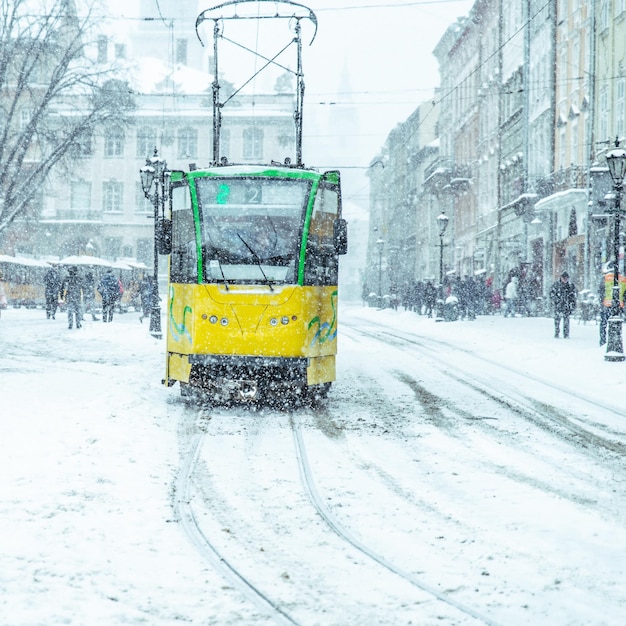In this detailed color photograph of a city street during a snowstorm, a bright yellow and green electric trolley is navigating snowy tracks. The trolley, adorned with green trim around the front and side windows, has a windshield wiper actively clearing snow. Its overhead electric cables are visibly connected to the power lines above. The snow is falling heavily, creating a magical yet somewhat obscured scene where pedestrians are walking or standing on snow-covered sidewalks. The tall, mostly gray high-rise buildings on either side, with occasional blue hints due to the snow, loom in the background. On the right-hand side, streetlights stand approximately eight feet tall, illuminating the snowfall. A large building with a snow-dusted leafless tree in the foreground enhances the wintry ambiance. The scene is bustling and serene, perfectly capturing a winter day in the city.